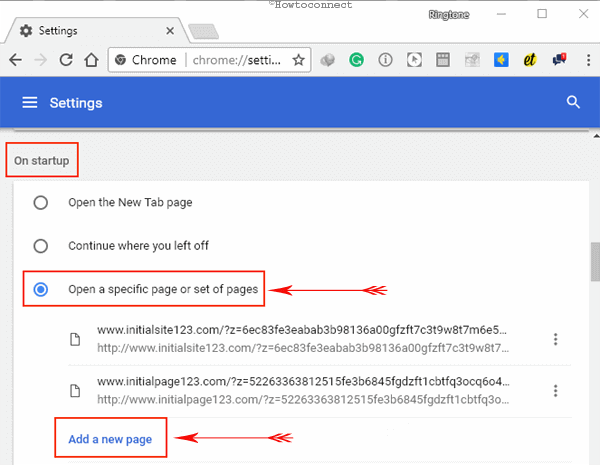The image displays a webpage, seemingly belonging to a company, providing instructions on how to connect. The main content area shows the Chrome browser's settings page, as indicated by the URL "chrome://settings" in the search bar. Various icons are visible at the top, including the Google logo. 

On the left, a navigation tab labeled 'Settings' is highlighted. The settings header appears on a blue bar with an hourglass icon to the far right. Directly below this header is a set of instructions under the "On startup" section, which offers three options: "Open the New Tab page," "Continue where you left off," and "Open a specific page or set of pages." These options are organized in a red-bordered box with a white background and have a red arrow pointing to the right side.

Within this instructions box, specific URLs are listed. The first URL shown is "initialsite123.com," followed by "www.initialpage123.com." Additionally, there's an option to "Add a new page," which is enclosed in a smaller white box with a red border and also features a red arrow pointing to its right.